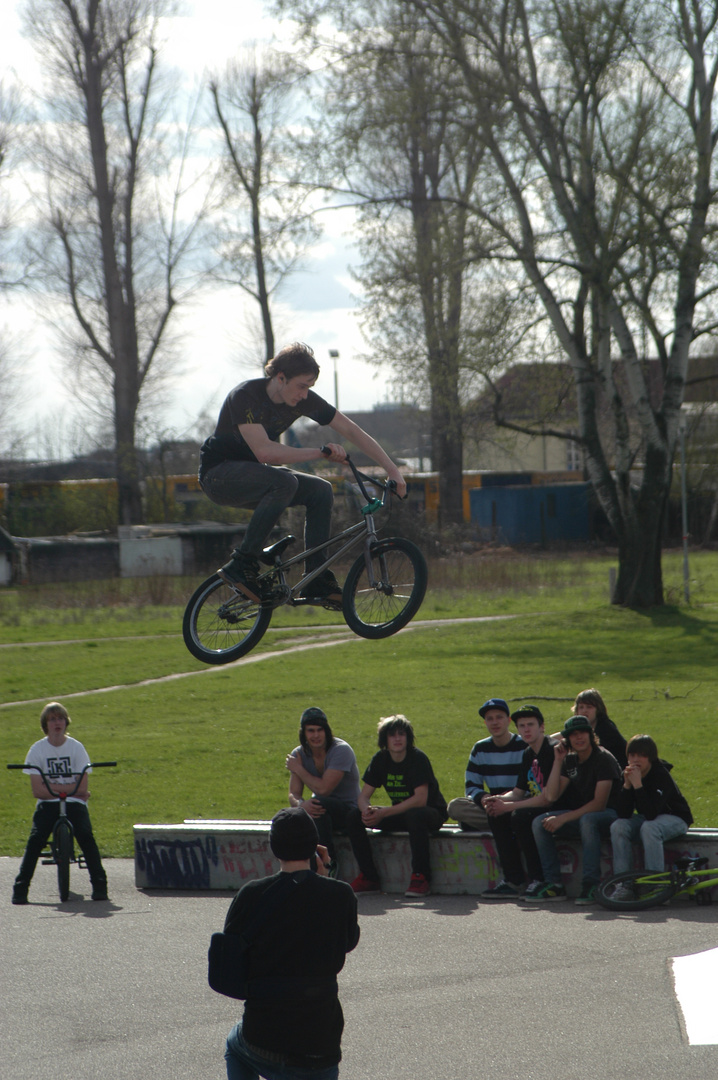In the photograph, a young male is captured mid-air performing an impressive bike or BMX trick, appearing to have just launched off an unseen ramp. He is approximately eight to ten feet above the ground, skillfully poised in a controlled position on his bike. The rider is dressed in a black t-shirt and long pants but notably lacks a helmet. Below him, eight teenage boys, predominantly white, are intently watching the stunt from a concrete area that appears to be part of a skate or dirt park. One of the observers, who seems to be filming, has his back toward the camera with his hand up to his face as if holding a camera. The audience is seated either on bikes or a curb-like structure. The scene's surroundings include patches of asphalt, grass, trees, and distant buildings, suggesting an open space suitable for performing such tricks, potentially near a school or park. The image lacks text but features a palette of colors including grey, black, blue, green, red, and white. The airborne rider occupies a slightly off-center position near the top of the frame, while the group of spectators is situated at the bottom, directing their gaze upward.